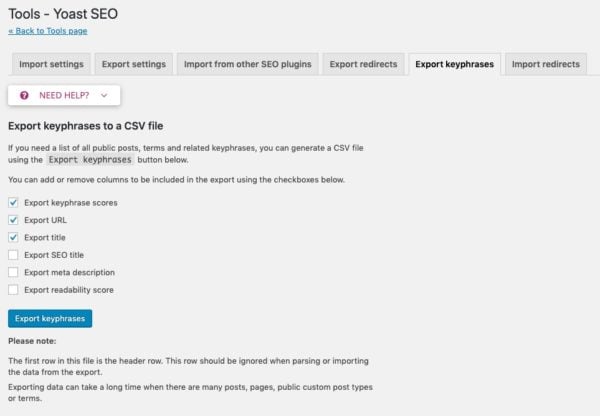The image depicts a section of a website interface with a minimalist design centered around Yoast SEO tools, primarily set against a white background. At the top of the page, there are two main menu options: "Tools" and "Yoast SEO." Below these options, a blue hyperlink titled "Back to Tools page" is visible. 

Directly beneath this link, a navigation menu is displayed, containing the following options: "Import Settings," "Export Settings," "Import from Other SEO Plugins," "Export Redirects," "Export Keyphrases," and "Import Redirects."

Further down the page, there is a help section labeled "Need Help?" Followed by an explanation and a button labeled "Export Keyphrases to CSV file." The accompanying explanatory text states: "If you need a list of all public posts, terms, and related keyphrases, you can generate a CSV file using the Export Keyphrases button below."

Next, there is a customizable export menu, which allows users to add or remove columns for the CSV export by using checkboxes. The available columns include: "Export Keyphrases," "Scores," "Export URL," "Export Title," "Export SEO Title," "Export Meta Description," and "Export Readability Score." Of these options, only the first three checkboxes are selected by default. 

Beneath the customizable columns menu is an option titled "Export Height Keyphrases," and finally, there is a note at the bottom of the page specifying: "Please note: The first row in this file is the header. This row should be ignored when parsing or importing the data from the export. Exporting data can take a long time when there are many posts, pages, public custom post types, or terms."